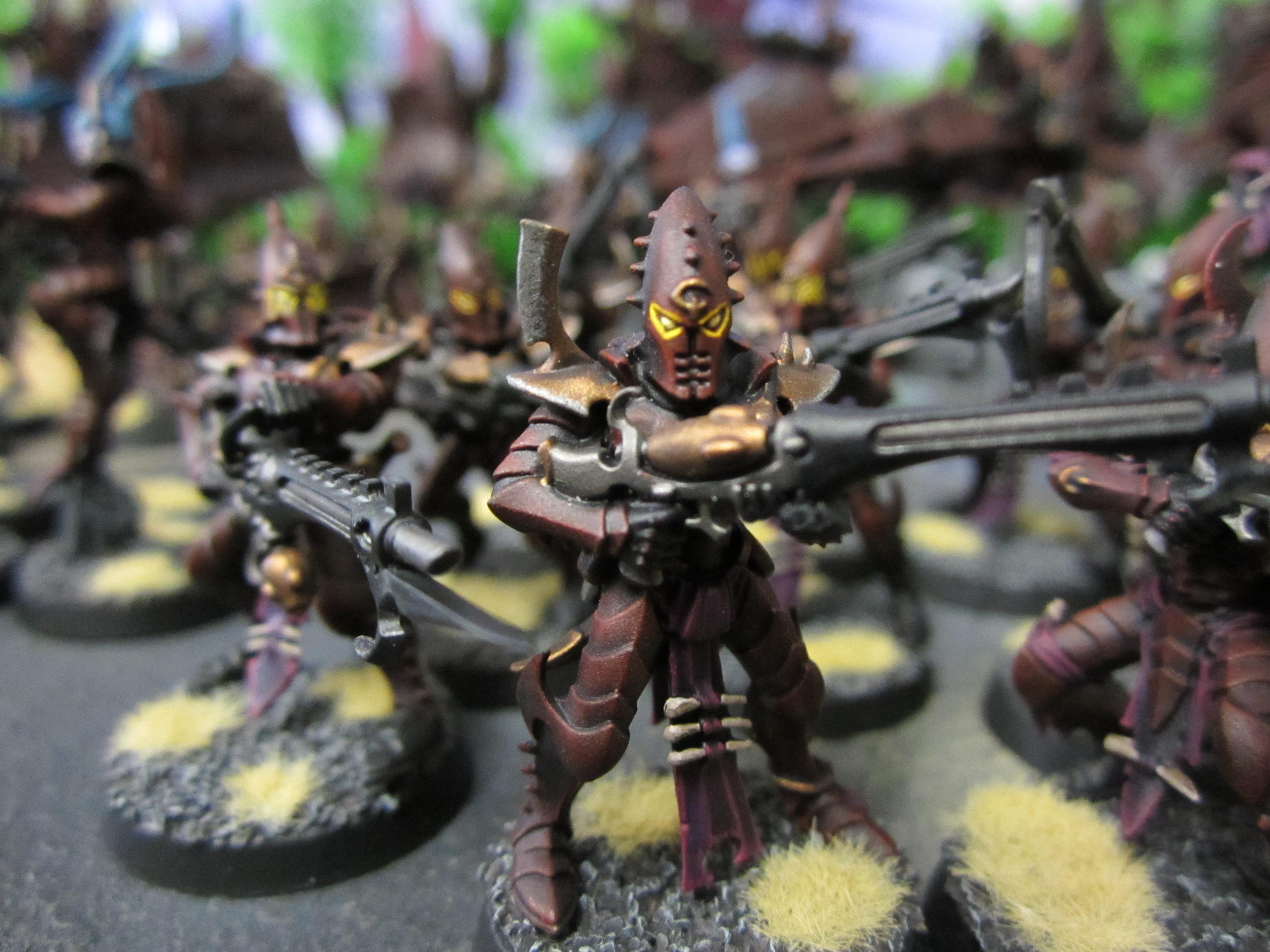The photograph is an up-close shot of numerous small, intricately painted figurines from the Warhammer science fiction universe, displayed on a black table. Amidst the many out-of-focus figures, the one in the center bottom is sharply in focus and draws immediate attention. This central figurine is a metallic red armored humanoid with a tall, cylinder-shaped helmet featuring three horizontal slits for the mouth and white eye holes bordered with yellow. The figure is wielding a long rifle-like weapon with a gold center and a black barrel. It stands firmly on a textured base resembling gravel, dotted with patches of brown grass. Noteworthy is the piece of cloth draped from its groin area, adorned with three small bones. The surrounding figures share a similar aesthetic, hinting at a unified army design, all equipped with matching garb and weaponry, albeit blurred. The background subtly shows hints of green and sky, adding depth to the scene.